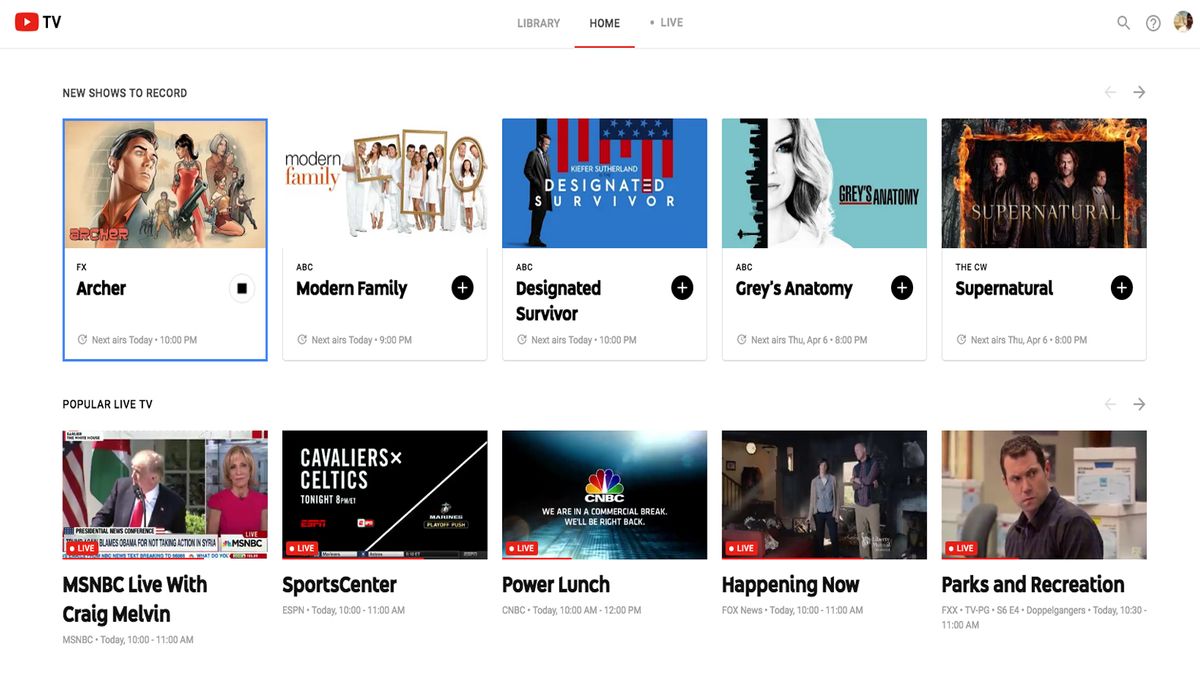The image displays the homepage of YouTube TV, characterized by its standard bright white background. In the top-left corner, the YouTube icon, featuring a red block with a white play button in the center, is prominently visible, with the word "TV" written in bold black letters beside it. At the top center, navigation options namely "Library," "Home," and "Live" are displayed, suggesting functionalities for accessing saved content, browsing recommended videos, and watching live TV, respectively.

On the top-right side of the interface, there is a search icon, a help or question mark icon, and a profile picture indicating the user's account. Below this section, there's a featured row titled "New shows to record," showcasing popular series such as "Archer," "Modern Family," "Designated Survivor," "Grey's Anatomy," and "Supernatural."

Additionally, at the bottom of the layout, there's a segment dedicated to live TV recommendations, highlighting shows currently airing live. These include "MSNBC Live with Craig Melvin," "SportsCenter," "Power Lunch," "Happening Now," and "Parks and Recreation."